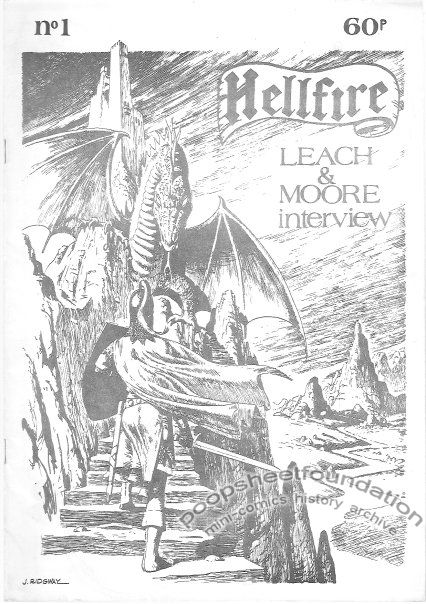The image features a vintage book cover or possibly the front page of a medieval-themed magazine. The cover is adorned with a detailed black and white illustration. At the very top left, the issue is marked as "No. 1," and the price "60p" is printed in black in the top right corner. Dominating the central part of the image is a dramatic scene: a knight, wearing a flowing cape and equipped with a drawn sword, shield, and helmet, ascends a stone staircase leading up a rocky crag toward a formidable dragon with two outstretched wings. Behind the dragon, a castle looms, adding to the medieval atmosphere. Text in ornate medieval font at the top right reads "Hellfire," with additional text below stating "Leech and Moore Interview." Farther below, in a slightly faded watermark style, the text "Poop Sheet Foundation Mini Comics History Archive" curves along the bottom of the image, blending into the background that also features distant mountains and a winding road. The artist has signed the illustration as Jay Ridgeway.